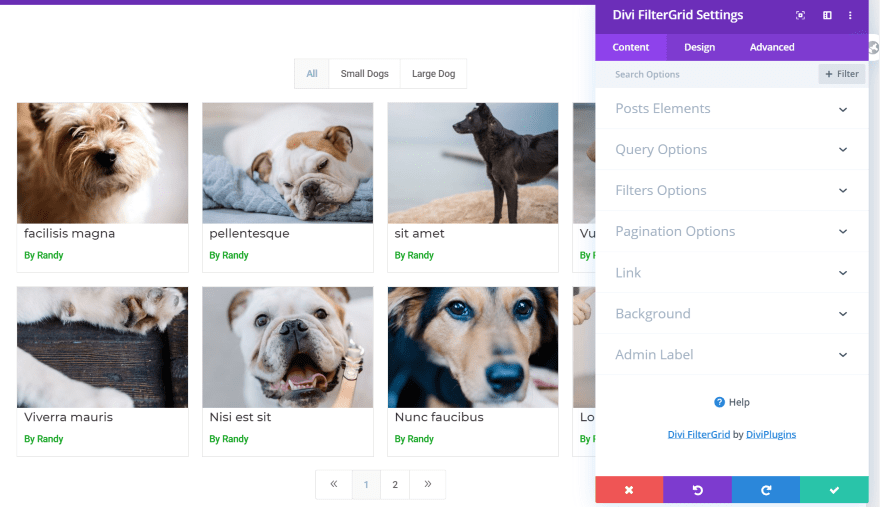The image showcases the user interface of a Divi Filter Grid settings panel, with a dark purple header appearing along the top. On the right side of the panel, the options "Content," "Design," and "Advanced" are listed. Below these, a series of settings categories are visible: "Search Options," "Filter," "Post Elements," "Query Options," "Filter Options," "Pagination Options," "Link," "Background," and "Admin Label," each accompanied by a drop-down icon on the right. At the bottom of the panel, there are helpful resources labeled "Help," "Divi Filter Grid," and "Divi Plugins."

On the left side of the image, there is a gallery display featuring six pictures of dogs, with a partial seventh image peeking in from the right side. Each photo is labeled with text: the top left image is titled "Facilities Magna by Randy," the top right one as "Pellentask by Randy," the middle left one as "Sit Amet by Randy," and the bottom left one is "Vivera Morris by Randy." The photo to the right of "Vivera Morris" is labeled "NCS Sit."